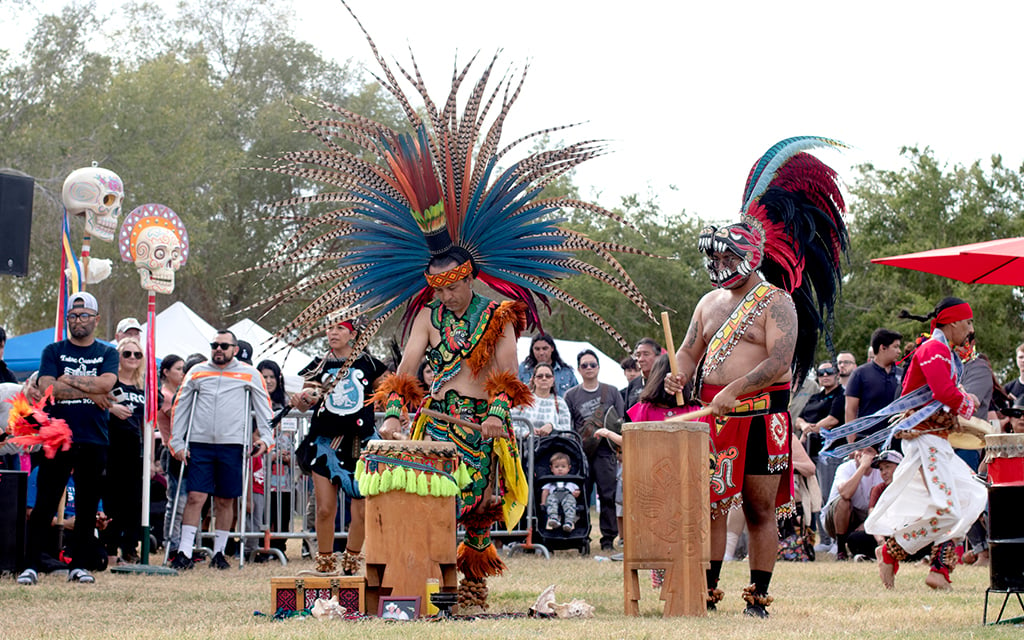The vibrant image captures a lively festival scene with a diverse crowd in the background. At the forefront, two men clad in elaborate Native American attire are passionately playing traditional drums adorned with leather and feathers. One man is dressed in vividly colorful clothing, including an orange headband and a headdress brimming with large feathers. His outfit features a spectrum of hues, including blues and greens, with feathers also embellishing his wrists. His companion, dressed primarily in striking red, wears a dramatic helmet-like hat resembling a dragon’s head, complete with sharp teeth and feathers protruding like a rooster's crest. A yellow sash adorns his tribal outfit. Behind them, an audience of various nationalities and ethnicities watches attentively. The backdrop features tall green trees, intricately designed skeleton head statues on poles, and glimpses of tents behind the spectators. Notably, one observer in the crowd appears to be injured, leaning on crutches as he enjoys the festivities.